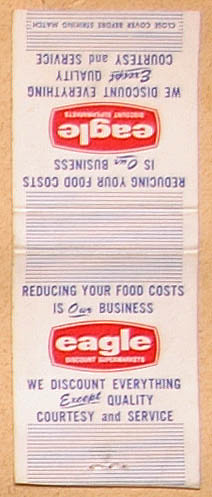This image depicts an open matchbook laid flat, exposing both the front and back sides in a mirror image arrangement, with the top portion upside down. The matchbook is primarily white, featuring blue text that reads, "Reducing your food costs is our business," followed by a red, rounded rectangular logo with large white letters spelling "EAGLE." Below "EAGLE," the text continues in blue with, "We discount everything except quality, courtesy, and service." The red logo also contains additional white text that is not fully legible but includes words like "discount" and potentially other descriptors. Surrounding the central text and design, there are blue stripes. The matchbook is attached to a brown cork-like board, suggesting it's secured with staples or pins. Note the top edge of the matchbook advises, "Close cover before striking match."